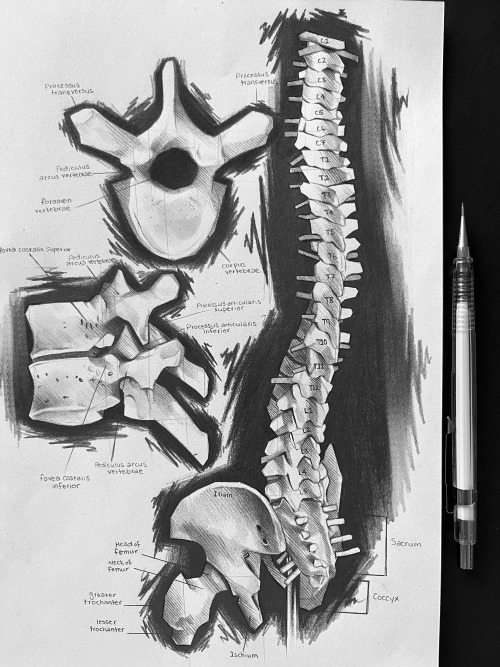This image is a detailed medical diagram of the spinal column, depicted on a rectangular piece of white paper with a black backdrop. The image, which measures approximately 5 inches high by 4 inches wide, features the spine prominently on the right side, with each vertebra numbered from the cervical (C1-C7) through the thoracic (T1-T12), lumbar (L1-L5), down to the sacral region and coccyx. Adjacent to the spine on the left, several bones including the hip bones and pelvis are also illustrated and labeled. Additionally, specific parts of the femur such as the head, neck, greater trochanter, and lesser trochanter are identified with lines connecting the labels to their respective parts.

The diagram extends to magnified views of individual vertebrae on the top left side, displaying detailed anatomy with labeled parts, although some text appears too small to decipher clearly. Positioned vertically to the right of the paper is a mechanical pencil with a clear casing and a silver tip, suggesting the drawing was hand-rendered by a skilled artist. The black text on the diagram is accented with a four-point underline directing attention to specific bones and features, enhancing the clarity and educational value of the illustration. The entire composition, executed in black and white, demonstrates a high level of precision and professional quality.